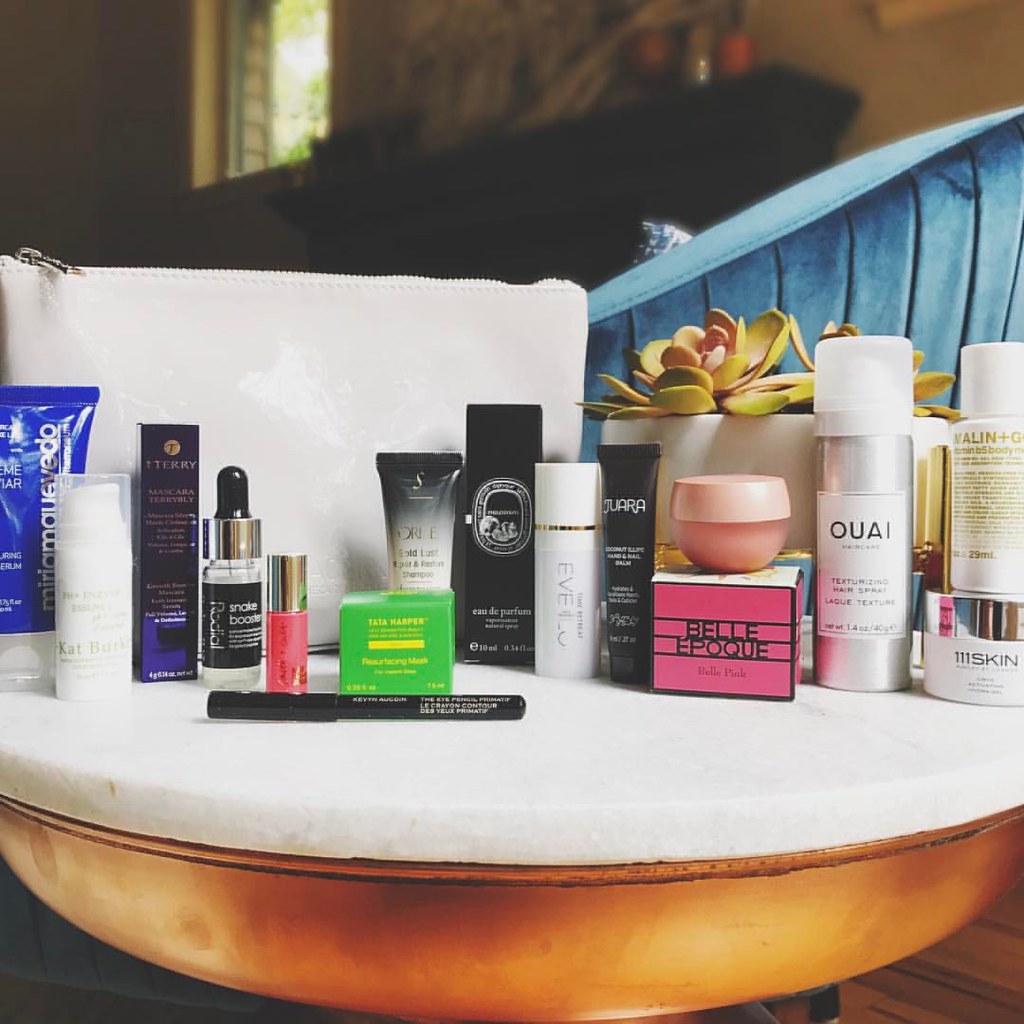The image showcases a meticulously arranged table adorned with various cosmetic items. The table itself features a sleek white, marble-like top paired with a striking gold-colored rounded base, adding a touch of elegance and intrigue to the scene. Positioned in front of a blurred background, the table appears to be set against what might be a piece of blue fabric, possibly hinting at the presence of a couch or bed nearby.

On the tabletop, an array of cosmetic products are neatly displayed. The assortment includes lotions, serums, and creams, each encased in vibrantly colored tubes and jars. Adding to the display is a white makeup bag with a zipper on top, standing upright behind the cosmetics. 

To the side, a small green succulent in a white pot adds a fresh and natural element to the arrangement. Among the visible product names are "Quora," "Belle Epoch," and "Tata Harper," indicating a diverse selection of high-end beauty products. The overall setting exudes sophistication and attention to detail, creating an aesthetically pleasing and functional space for beauty enthusiasts.